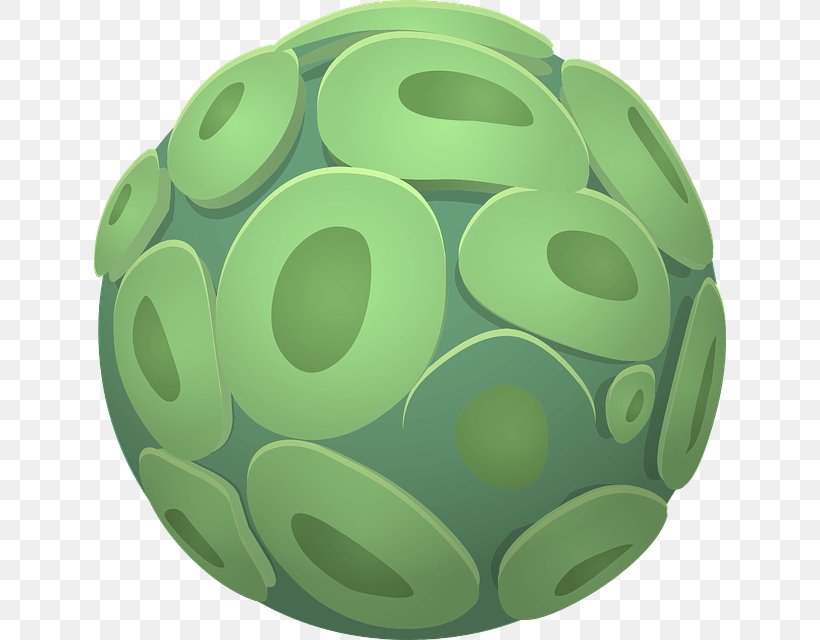The image features a piece of graphic art set against a small, alternating checkered background of light gray and white squares. Dominating the center is a large, teal-colored spherical object adorned with various circular and oval shapes. These shapes, resembling bubble letter "O"s or donut-like forms, are predominantly light green with darker green centers, slightly raised and interconnected in an intricate pattern. The sphere's overall hue is darker than the central portions of these green shapes, giving it a rich, almost globe-like appearance. Despite the intricate design and patterns on the sphere, the checkered background, though detailed, becomes a subtle backdrop to the visually compelling central sphere.